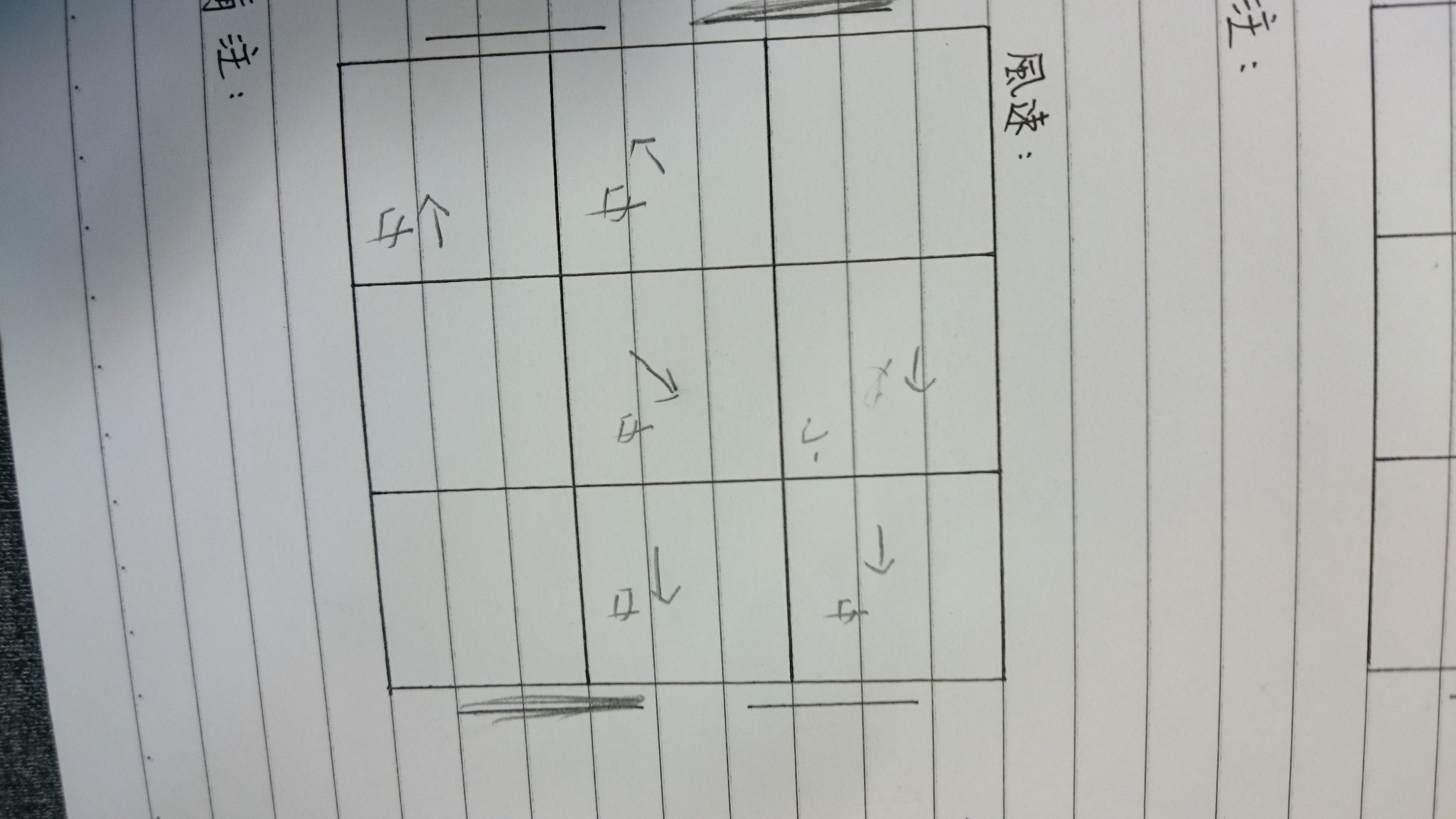The image depicts a detailed pencil drawing on a large sheet of white paper, featuring a series of white lines running horizontally across the entire surface at half-inch intervals. Central to the composition is a large, dark black square, subdivided into six smaller squares arranged in two rows of three. Each smaller square contains an intricate design characterized by an 'X' with a line intersecting in the middle, adorned with an arrow either pointing up or down.

Adjacent to the edge of the paper, there is evidence of preparation for another set of designs, with hints of additional squares partially visible. Specifically, the middle smaller square within the large central one displays the same 'X' design, accompanied by an upward-pointing arrow. The bottom middle square, along with two other bottom squares, feature designs with arrows pointing downward.

An area below the central drawing is marked by a dense, black scribble spanning about nine or ten strokes. Additionally, the right side of the paper includes a singular horizontal line, paralleled by a similar line at the top. Both these lines are accentuated by scribbled areas on their right sides, referenced by nine repeated back-and-forth strokes.

Interspersed throughout the drawing are inscriptions resembling Chinese or Japanese characters, contributing to the overall complexity of the piece. Two distinct symbols are notable: one located on the side of the main central square and another situated just before the inception of a second prominent square structure.

Overall, the artwork combines geometric precision with intricate detailing, underpinned by both Western and Eastern aesthetic elements.